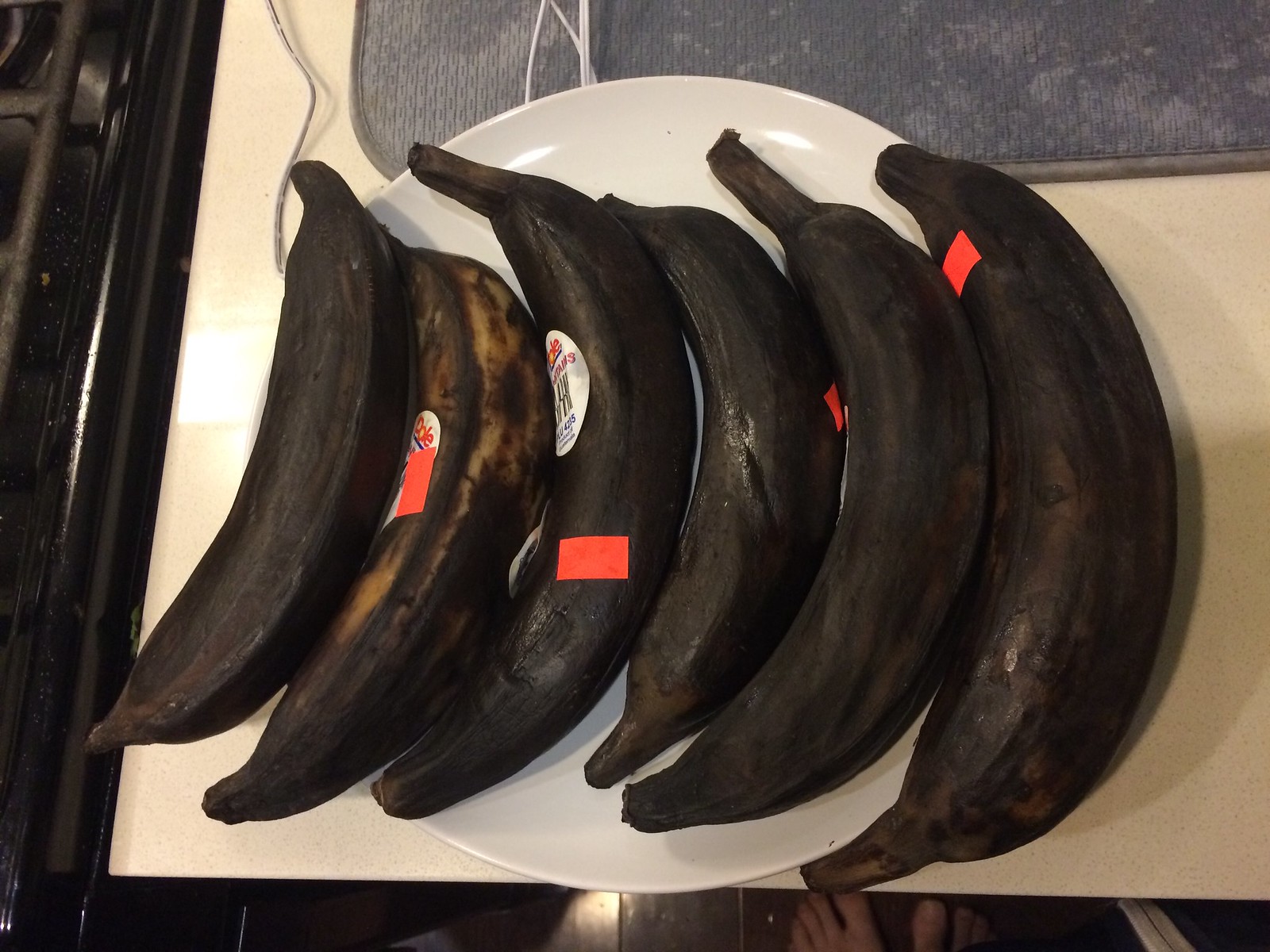This is a detailed color photograph taken indoors, capturing a close-up, overhead view of a white ceramic plate positioned on a white countertop or table. The plate holds six bananas that are extremely black and thoroughly overripe, their peels appearing almost rotten. Positioned with their tops pointing towards the top of the image and slightly curved to the right, the bananas are adorned with both dull product identification labels and bright red or orange rectangular clearance stickers, signaling their reduced price status. All but one of the bananas are uniformly black, with the exception of one that shows faint yellow streaks amidst the darkness. Visible to the left is a hint of a dark appliance, likely an oven, and at the top of the frame, there's a glimpse of a blue kitchen towel or mat, slightly below the plate. The lighting highlights the glossy surface of the plate and the neglected state of the bananas, offering a stark contrast against the clean, white background.